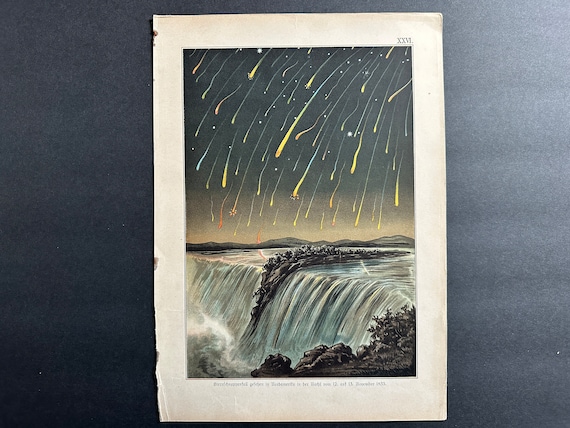This is a detailed depiction of a surreal photograph of a painting hanging on a very dark charcoal gray wall, which almost appears black due to its intense shade. The painting is framed with a white paper-like border, adding a stark contrast to the dark background. 

The artwork itself captures a fantastical scene of a waterfall at night. The water in the painting is rendered with impressive realism, cascading over the edge of a cliff, flanked by rocky edges and sparse vegetation, including some trees and plants. What sets this piece apart and leans into the surreal is the addition of vibrant, colorful elements that appear like shooting stars or fireworks. These streaks, painted in hues of yellow, blue, red, and purple, descend from the sky towards the ocean, creating a vivid, dynamic scene. In the background, majestic mountains rise, grounding the scene with a touch of natural grandeur.

On the right-hand side of the painting, the letters "XX" are visible, while at the top, the text "XXXL" is noted. There is also some writing at the bottom of the painting, though it's too small to discern clearly. The entire composition, while inspired by the realistic portrayal of natural elements like water and rocks, is enhanced by the dramatic, possibly celestial occurrences, blurring the line between reality and the fantastical.